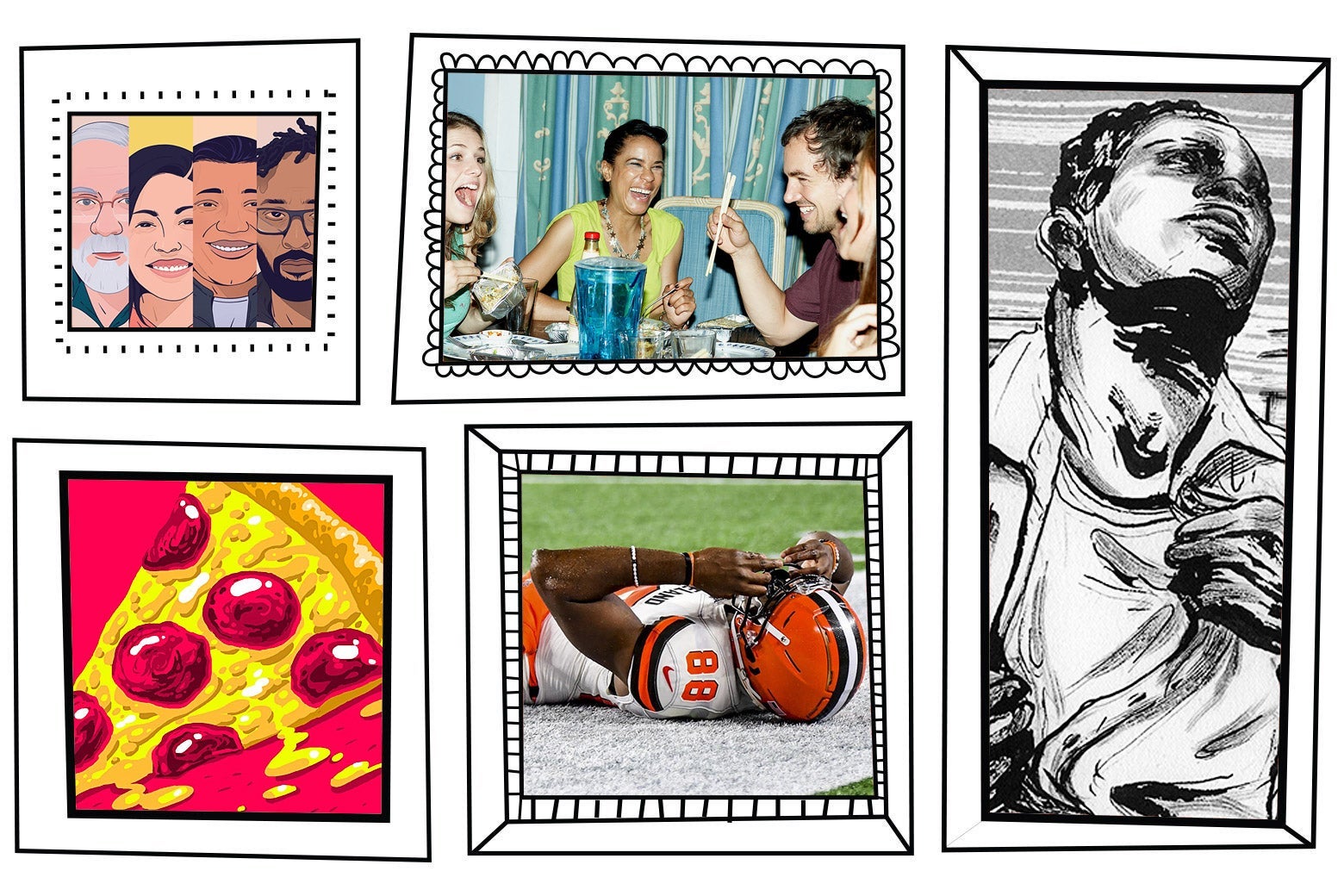The image is a detailed collage of five smaller pictures, each enclosed in hand-drawn frames with distinct borders and varying artistic styles. The top left frame features an illustrative drawing of four faces, each partially cropped. The group includes an old man, a middle-aged woman with dark hair, a middle-aged man with a darker skin tone, and a black man with glasses and a beard. Adjacent to this, in the top middle, is a vivid photograph of four people joyfully laughing and eating at a table against a blue background. Far right, a striking black-and-white pencil sketch depicts a man in a t-shirt and a button-down shirt, dramatically pulling open the button-down while looking upwards. In the bottom center frame, a vivid photograph captures a black football player lying on the field with his hands covering his face, wearing an orange helmet and a white jersey with orange and black details. Lastly, in the bottom left corner, an illustration showcases an enticing slice of pepperoni pizza with ooey-gooey cheese, set against a red background. The collection of images, each distinct in content and style, offers a dynamic visual experience akin to viewing a series of pictures hanging on a wall.